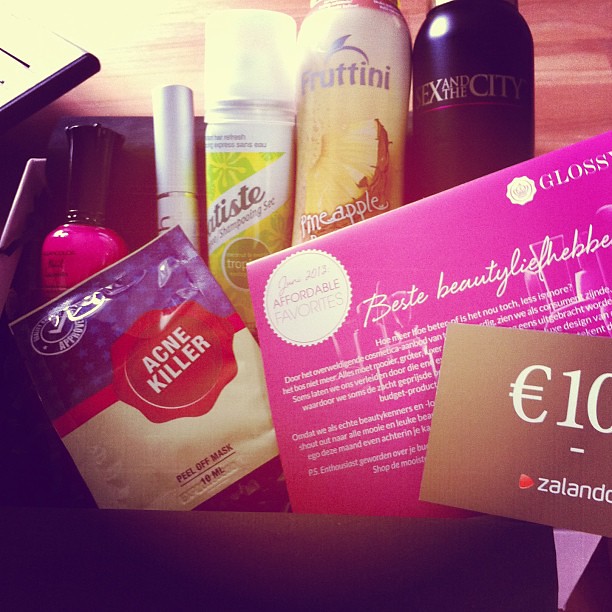This image, likely an Instagram post with high contrast and a somewhat grainy quality, depicts a diverse assortment of beauty and self-care products arranged on what appears to be a wooden table. On the left, there is a small bottle of pink nail polish beside a packet labeled "Acne Killer." Prominently featured in the middle is a Frutini product, identifiable by a picture of a pineapple on it and the brand name clearly displayed. Nearby, there is another spray bottle possibly used for shampooing, as the blurry label suggests. A silver cylindrical item, possibly lipstick or an eyelash container, is also present.

Towards the right of the image, a large pink box or packaging marked "Affordable Favorites" stands out, with a logo reading "Gloss" at the top right corner. Draped over this box, there's a €10 gift card. Another notable item is a black bottle with the "Sex and the City" logo, indicative of a fragrance or body spray, positioned at the far right. Adjacent to these items is a yellow canister whose specific contents are unclear.

In front of the pink box is a sign that reads "£10," possibly relating to the price. Additionally, details suggest there is some descriptive card, possibly explaining the contents of the beauty package, lying near the lower right side of the image. The entire arrangement seems curated for a visually appealing display, highlighting a variety of beauty essentials.